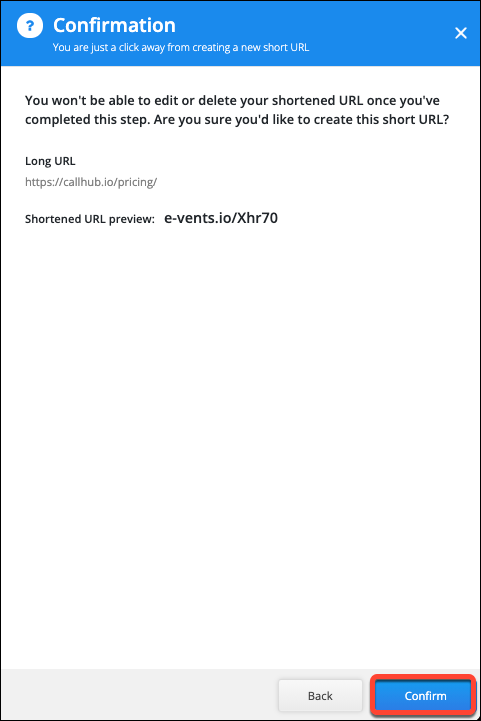Screenshot Description:

The screenshot is enclosed by a thin black border. The top section, about an inch and a half tall, features a rich, deep blue color. In the top left corner, there's a white circle containing a blue question mark. To its right, prominent bold lettering spells out "Confirmation" with smaller text below stating, "You are just a click away from creating a new short URL." The term "URL" is all capitalized. On the far right of this blue section, there's a white "X" icon.

Below this blue header, the background is predominantly white. About an inch below the header on the left side, bold black text reads: "You won't be able to edit or delete your shortened URL once you've completed this step. Are you sure you'd like to create this short URL?"

Further down, there is a slight gap before more black text appears: "Long URL." Underneath this, the URL "https://callhub.io/pricing/" is displayed. Below this URL, smaller black text labels it as the "Shortened URL preview" with the shortened version "https://evince.io/xhr70" shown directly beneath it.

A large gap of white space extends towards the bottom of the screenshot. Finally, at the bottom, there is a lighter gray background. In the bottom right corner, a blue rectangular tab with a thick red border contains the word "Confirm" in white text. To its left, within a lighter gray tab, the word "Back" is written in black text.